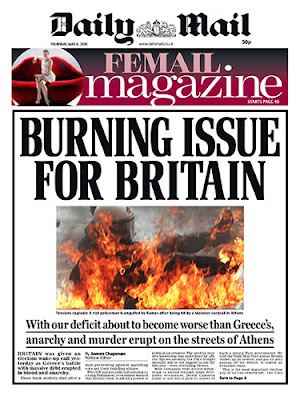This detailed caption provides an exhaustive description of the front page of the Daily Mail newspaper, specifically from the Female Magazine section, dated Thursday, May 6, 2010, with a cover price of 50 pence.

**Descriptive Caption:**

The front page of the Daily Mail, dated May 6, 2010, prominently features its Female Magazine section. The header displays "Daily Mail" with the date and price of 50 pence clearly indicated. The section title "Female Magazine" stands out in an elegant, bold font set against a dark maroon background.

Dominating the page is a dramatic, large photo capturing a chaotic and urgent fiery scene with intense flames and smoke. The sense of turmoil is palpable, with a figure in the background appearing to be engulfed in flames. The situation depicted reflects a crisis scenario.

Above the image, in large, bold capital letters, the headline "Burning Issue for Britain" grabs attention. Below this, a poignant subheading reads, "With our deficit about to become worse than Greece's, Anarchy and murder erupt on the streets of Athens," underscoring the severity of the situation. This narrative is italicized and credited to journalists James Chapman and Robert Hardman.

The front page employs dramatic visuals and bold typography to highlight and emphasize the pressing financial and social issues, effectively conveying the potential consequences.